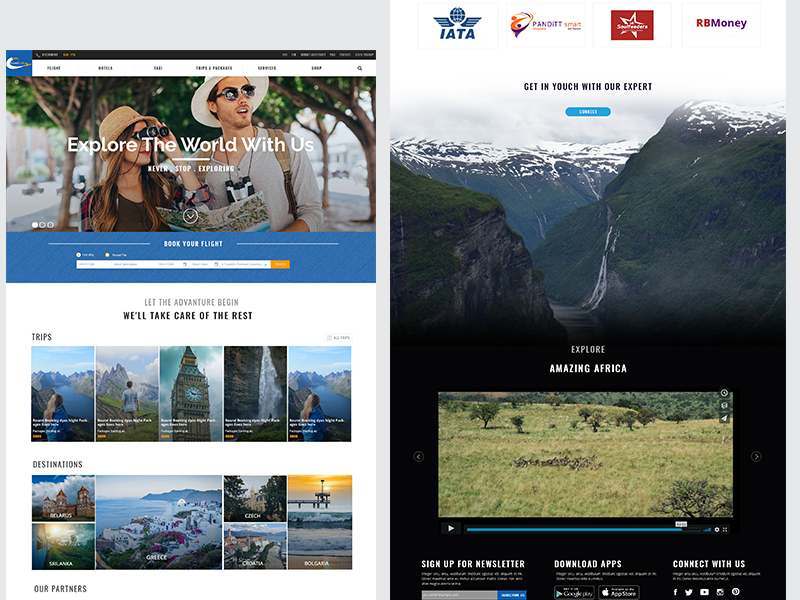The image shows two side-by-side screens of a travel website. 

**Left Screen**: The main section features a large banner depicting a man in sunglasses and a hat, and a woman with binoculars and a hat, both gazing towards the right while holding a map. The man also has binoculars hanging around his neck. Superimposed on the photo, white text reads "Explore the World with Us" and below it, "Never Stop Exploring." Further down, a blue banner with white text prompts users to "Book Your Flight," followed by a search bar for various travel inquiries. Beneath this, a white background holds additional white text stating, "Let the adventure begin, we'll take care of the rest," accompanied by options for different trips and destinations to choose from.

**Right Screen**: This screen displays a picturesque mountain landscape with the text "Get in touch with our get in yutch with our expert," where "touch" is misspelt as "yutch." Below this text, there is a clickable blue button. The top of the screen showcases logos of various businesses, likely sponsors of the website. At the bottom, a video awaits viewers with the label "Explore Amazing Africa," showing a captivating landscape from the continent and marked with a play button. 

The layout and design aim to inspire and assist users in planning their next travel adventure, providing a blend of visual appeal, interactive elements, and accessible information.